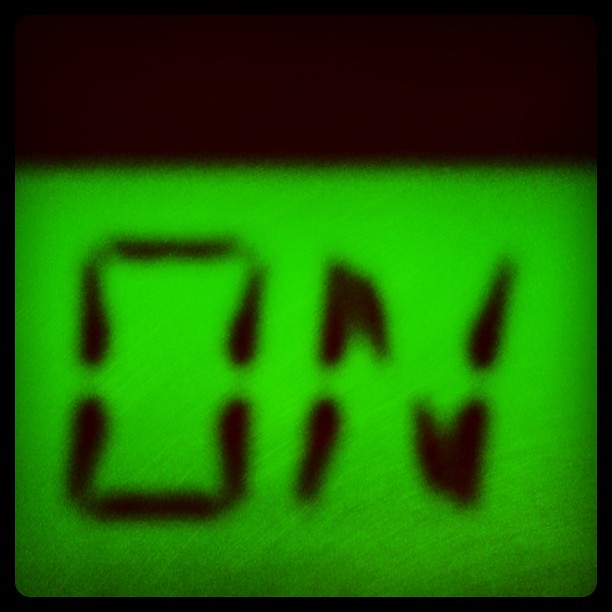The image is a close-up of a digital screen, possibly from an appliance or alarm clock, displaying the word "ON" in large black letters. The screen itself is predominantly neon green, with slight variations in shade, being lighter and brighter in the center and darker on the edges. The letters "O" and "N" are pixelated, featuring noticeable gaps, as typically seen in digital displays. The top third of the image is a solid black background, contrasting sharply with the green screen, which occupies most of the image and is slightly blurry, indicating poor camera quality.